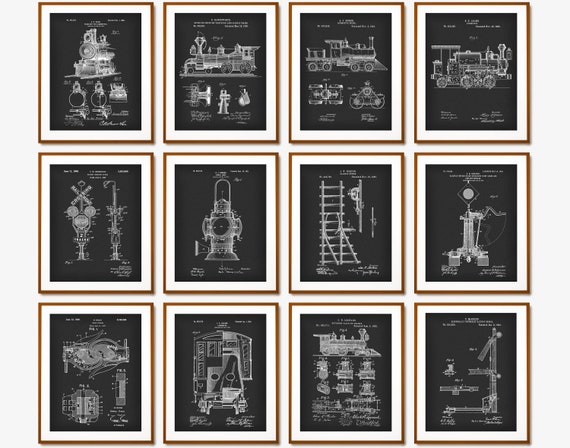The wall displays a neatly arranged collection of 12 framed artworks, positioned in a grid of four rows across and three down. Each piece is a vertical rectangle, encased in a simple wooden frame with a white mat background, highlighting the black backdrop of the images themselves. The artworks are detailed, black-and-white diagrams and artist renderings, all centered around the theme of trains. This collection includes various perspectives and components of trains: side views, front views, detailed examinations of wheels, train stops, switch posts, a lantern light, and a train crossing sign. Some images are intricate diagrams with labeled parts, making the mechanical workings and connections of the train elements clear. The presentation is cohesive and methodical, giving an almost educational insight into different aspects of locomotive technology and infrastructure.